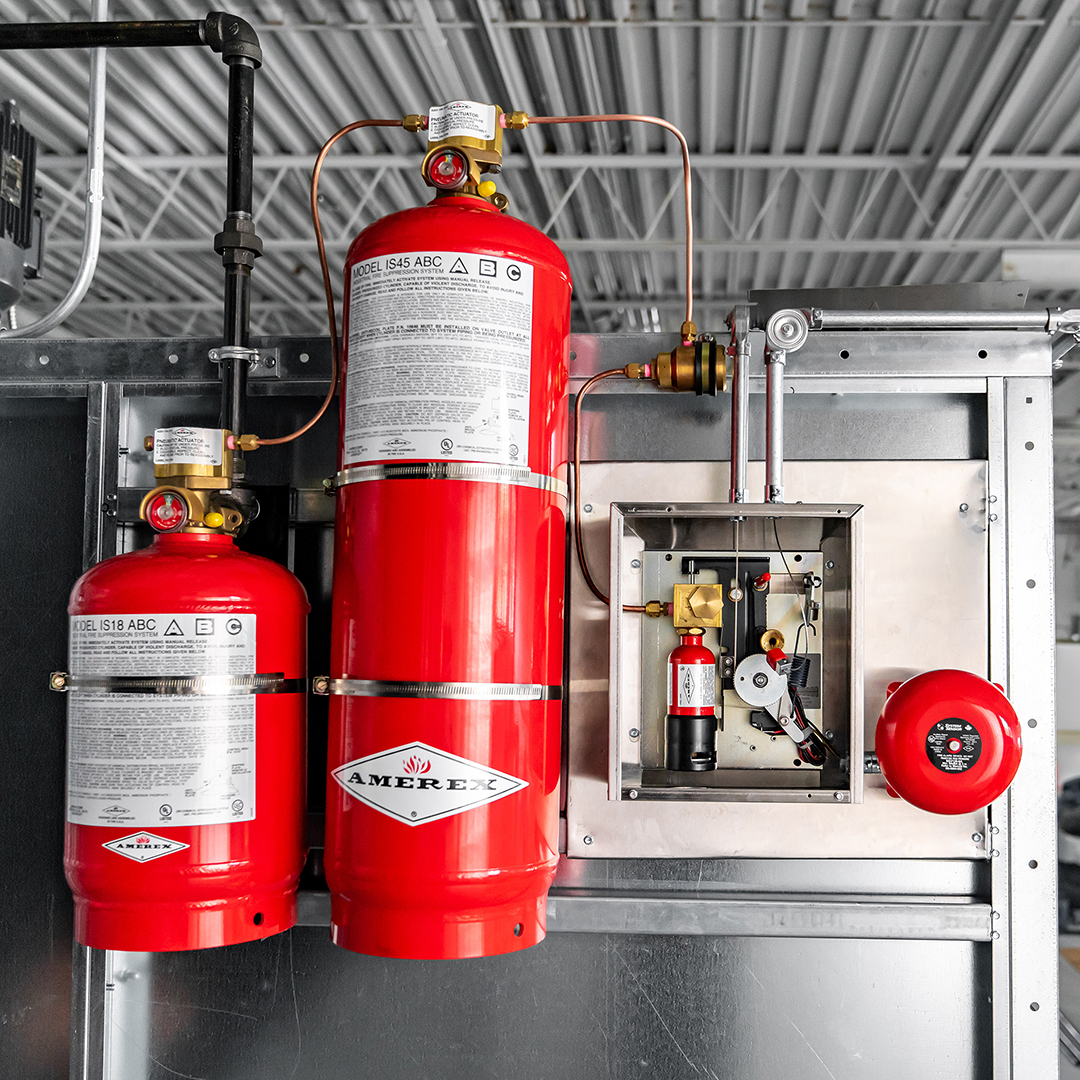The image captures the interior of a gray industrial building, likely a warehouse or manufacturing facility, characterized by its corrugated steel ceiling with white-ish paint. Prominently displayed in the foreground is a complex fire suppression system. The system features multiple interconnected red pressurized canisters labeled "Amerex," adorned with a black label that includes the company's name and flame symbols. The setup includes both a larger and a smaller canister, linked by copper tubing and pipes that run to the left side of the image. An open metal box reveals intricate mechanisms, including a gauge with a red dial, various connected pipes, nuts, bolts, and a timer with gears. A red alarm bell sits to the right of the canisters, complementing the industrial aesthetic.